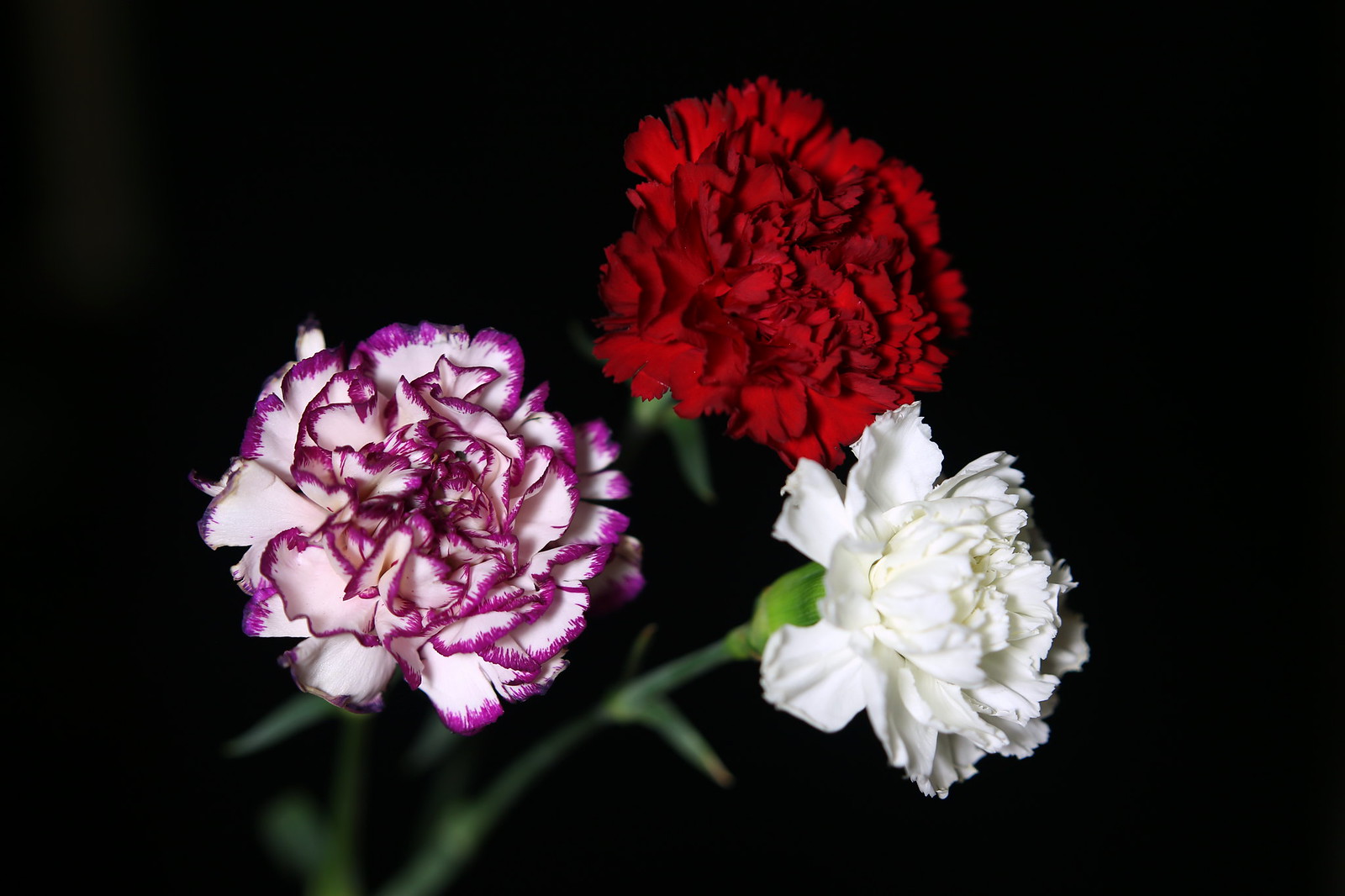A close-up photograph showcases three blooming carnations against an entirely black background, with their green stems trailing down to the left and bottom of the image, blurred and out of focus. The carnation at the top is a deep, regal red, while the one at the bottom right is a bright white. The third carnation, positioned on the left, is a striking variegated bloom with primarily white petals that transition to magenta at the edges. We look directly into the center of the magenta-edged carnation, with the red and white ones slightly facing to the right. The flowers, known for their many ruffled petals, are the clear focal point of the image, standing out starkly against the dark, featureless background.